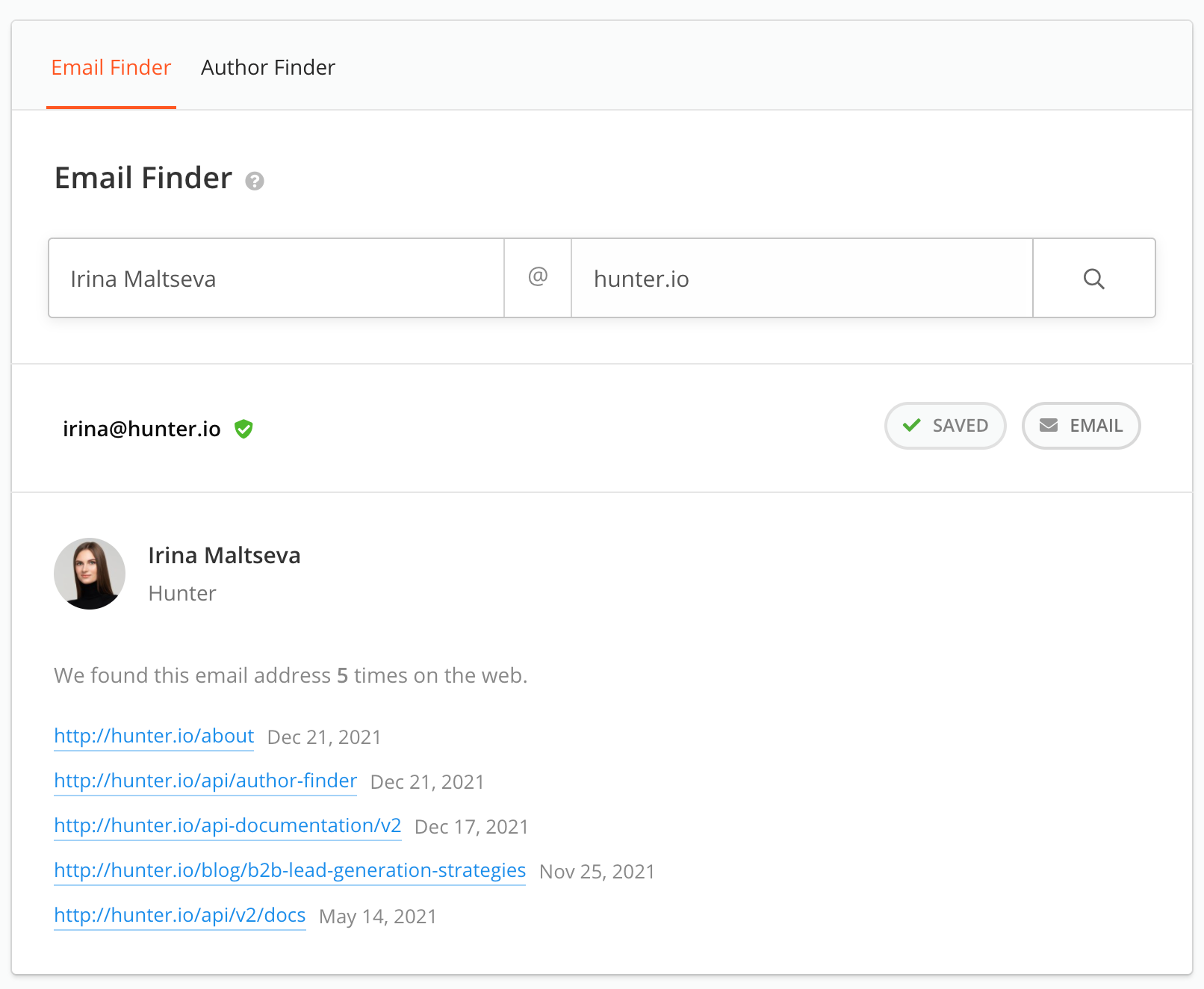This screenshot showcases a webpage designed for searching specific email addresses on the internet, featuring a layout with distinct visual and functional elements. The page has a clean white background, topped with a light blue navigation bar containing two selectable tabs: "Email Finder" (highlighted in red and underlined, indicating selection) and "Author Finder."

Below this navigation bar, the title "Email Finder" is displayed alongside an information icon (a circle with a question mark) for accessing frequently asked questions. Beneath the title, there is an input bar where users can enter part of an email address, pre-structured to include the "@" symbol, followed by an option to complete the domain after typing the user's name. A search icon (magnifying glass) is present for initiating the search.

In the specific example shown, the email "irina@hunter.io" is being searched. The results section features a green shield with a checkmark, followed by two interactive pill-shaped buttons: "Saved" (with a green checkmark) and "Email" (with an envelope icon), providing quick actions for saving or emailing the found address.

The entry displayed includes an avatar of a fair-skinned woman with long brown hair, wearing a black turtleneck, identified as Irina Maltseva. Her email was located five times on the web by the service. The details include the source URLs in blue font and the dates found in gray font, adding an additional layer of authenticity and traceability to the provided information.